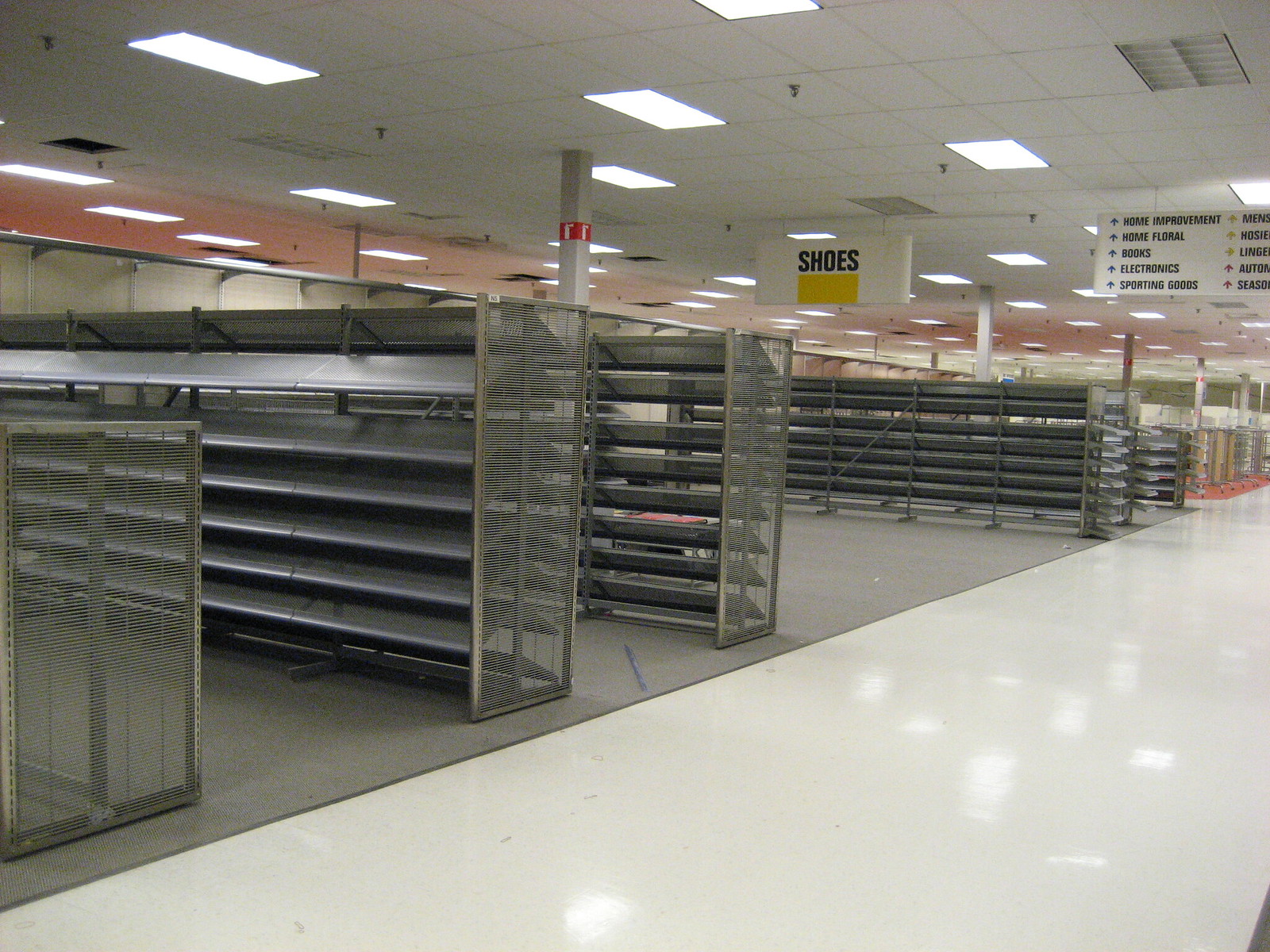This photograph captures the interior of an unspecified retail store, potentially a department store, characterized by its stark emptiness. The floor is predominantly covered in white tiles, commonly found in retail settings, which transition into a gray carpeted area on the left side of the image. The store features an array of metal shelving units, each consisting of six or seven shelves, all devoid of merchandise.

Toward the end of these shelving units, a screening material is visible, contributing to the industrial aesthetic of the store fixtures. The ceiling is a classic drop ceiling design, equipped with large, recessed lighting panels that illuminate the space.

In the background, a prominent white sign with black lettering lists various departments such as "Home Improvement," "Books," "Electronics," accompanied by arrows indicating the directions to each department. This sign is located on the back right side of the store. Closer to the middle right, another white sign with the word "Shoes" in bold black letters hangs from the ceiling, accentuated by a small yellow rectangle beneath it.

Additionally, a few pillars are scattered throughout the store, each featuring a red sign at the top, further contributing to the store’s wayfinding system. Despite the detailed layout and signage, the complete lack of merchandise imparts an eerie, abandoned atmosphere to the scene.